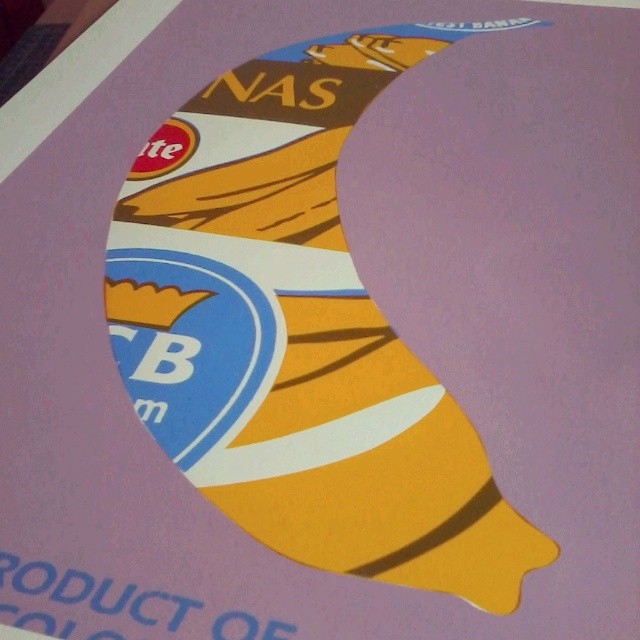This image depicts a purple box with a white edge on the upper left side and some brown visible in the corner, suggesting it might be sitting on a brown desk. The bottom left corner of the box has blue, capitalized text that partly reads "PRODUCT OF," although some of the bottom letters are not visible. The most prominent feature of the image is a cutout in the shape of a banana that is filled with various colors and images. The banana shape is primarily yellow with brown stripes along the bottom, and it contains smaller images of bananas. Across this banana cutout, there is a blue and light blue shield featuring a gold crown, with part of a white letter "B" visible. There's also a recognizable piece of a red background outlined in gold, likely indicating part of the Del Monte logo, with the letters "TE" readable.